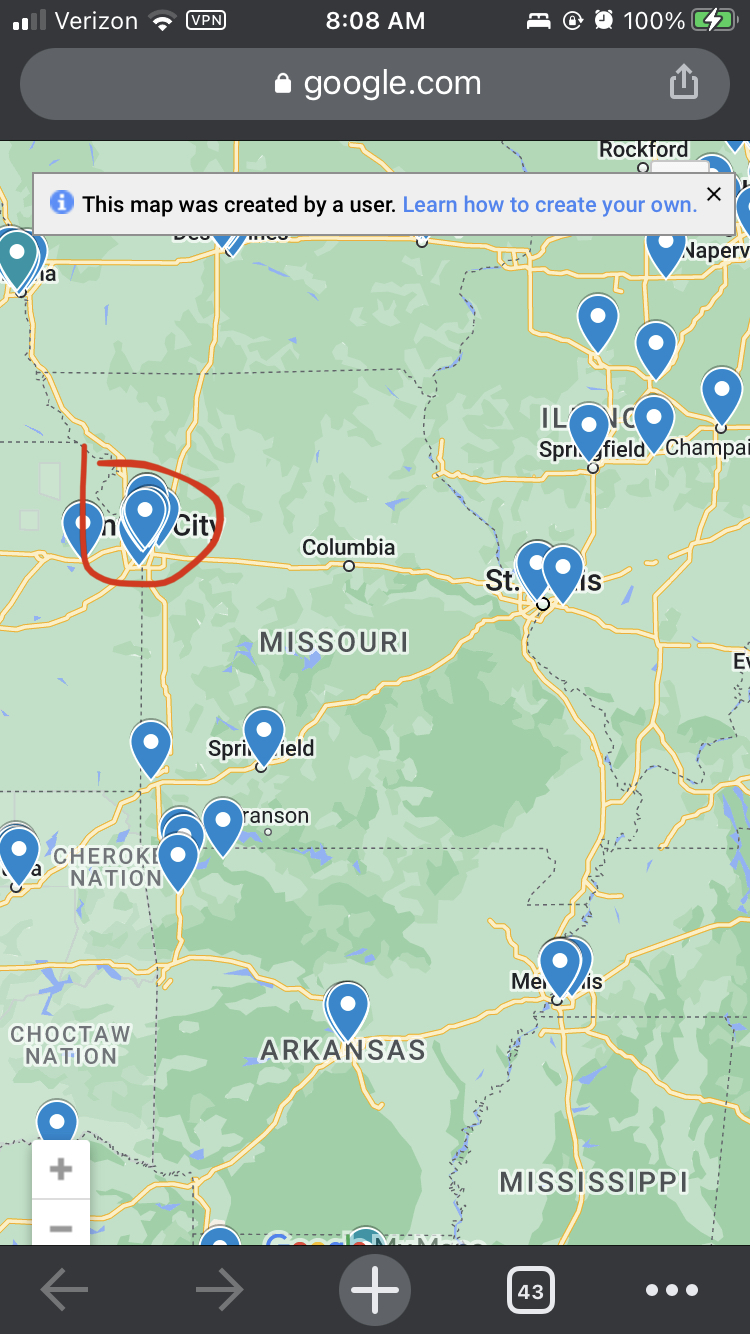The image depicts a screenshot of a Google Maps interface displayed on a smartphone. The top of the screen shows various indicators, including two bars of cell service labeled "Verizon," two bars of Wi-Fi signal, a VPN indicator, and the time, 8:08 AM. Additionally, there are icons representing a bed, a charging status, and an alarm clock, along with a green battery icon showing a full charge of 100%.

Below the status icons, the search bar reads "Google.com." The map mainly highlights the Ozarks area and encompasses parts of Missouri, Illinois, Arkansas, Mississippi, and their surrounding states. A white bar within the map states "This map was created by a user," followed by a blue hyperlink encouraging viewers to "learn how to create your own."

The map is populated with numerous blue pins marking various locations. Notable concentrations of pins are seen in Memphis, Little Rock, Tulsa, the Branson to Bentonville area, Springfield (Missouri), St. Louis, Springfield (Illinois), Champaign (Illinois), and the Chicago area. A significant cluster of pins is encircled in red around the Kansas City area.

At the bottom of the screen, a gray bar contains navigation buttons, including a back button, a forward button, a plus button, an indicator showing 43 open apps, and a three-dot hamburger menu for additional options.